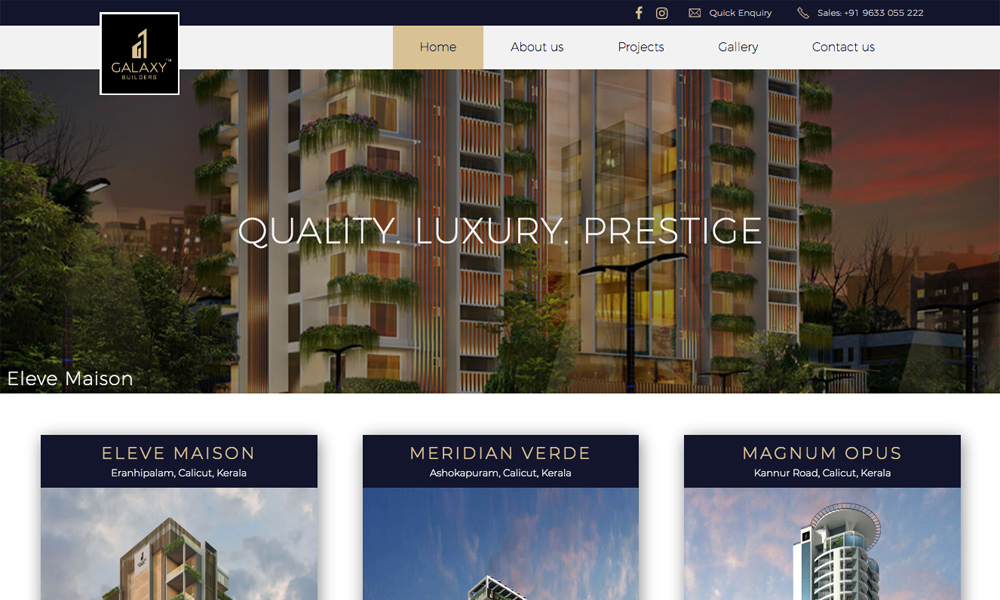Screenshot of Galaxy Builders Hotel Website:

The image appears to be a screenshot from the Galaxy Builders hotel website, characterized by a sleek and professional layout.

**Header:**
- **Logo:** Galaxy Builders in the upper left corner
- **Navigation Tabs:** Home, About Us, Projects, Gallery, Contact Us
- **Social Media Icons:** Facebook, Instagram, and an email icon in the top right corner
- **Miscellaneous:**
  - A "Quick Inquiry" logo is also visible
  - Phone number displayed: 919-633-055-222

**Main Content:**
- **Center Image:** Side view of an elegant building, with overlaid text stating "Quality, Luxury, Prestige"
- **Bottom Left Text:** "Eleve Mason," possibly the name of the building or project

**Thumbnails at Bottom:**
1. **First Image:** Partially cropped, labeled "Eleve Mason, Aaron Hypalum, Calicut, Kerala"
2. **Second Image:** Labeled "Meridian Verde, Ashokapuram, Calicut, Kerala"
3. **Third Image:** Labeled "Magnum Opus," also located in Ashokapuram, Calicut, Kerala

The overall layout is designed to highlight the quality and prestige of the properties offered by Galaxy Builders, focusing on their luxury projects in Calicut, Kerala.